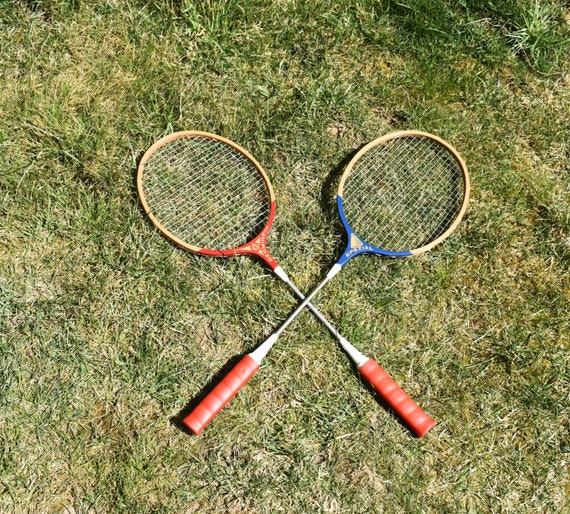The photograph shows two tennis rackets positioned diagonally, intersecting to form an X shape on a green grass background, which includes a few patches of yellow. Both rackets feature wooden frames, an unusual choice compared to the more common carbon materials used today. The racket on the left has a red base and a light brown border, while the racket on the right has a blue base and similar light brown bordering. Each racket sports light white twine across its head. Distinguishing the handles are red bindings or tape, a common feature on both. The overall arrangement draws attention to the contrasting yet complementary colors and materials of the rackets, all set against the lush, green grass.